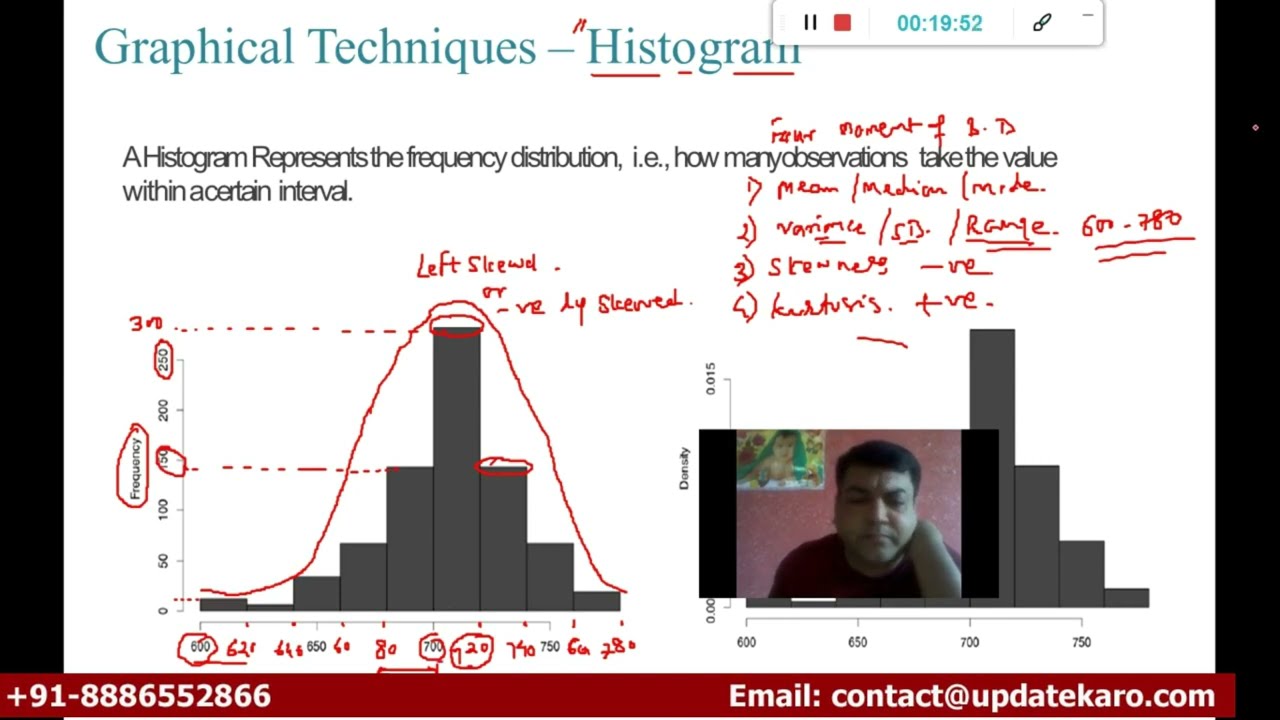The image is a horizontally aligned rectangular screenshot that resembles a PowerPoint slide, surrounded by thick black borders on the sides and a red border at the bottom. The bottom right corner of the red border contains the email "contact@updatekaro.com," and the bottom left corner shows the number "+91-888-655-2866."

At the top of the white background slide in teal Times New Roman font, the title reads, "Graphical Techniques - Histogram." Directly below, the text explains, "A histogram represents frequency distribution, i.e., how many observations take the value within a certain interval."

On the left side of the slide, there is a graph where the x-axis is numbered, though partially obscured by red handwritten annotations, and the y-axis is labeled "frequency," ranging from 0 to 250, with 150 and 250 circled. Words like "left-skewed" or "very skewed" are scribbled around it.

On the right side, another graph is present, labeled with a y-axis that reads "density." Overlapping this chart is an image of a man with dark hair who appears to be of Indian descent, looking down with his elbow on his head. The background of his photo is brown. 

The slide contains red handwritten notes throughout, demonstrating annotations which seem hurried and difficult to read. In the upper right corner, there is a pause and stop button icon, along with a timestamp "00:19:52," suggesting this could be a paused video or a streaming presentation, possibly an educational lesson.